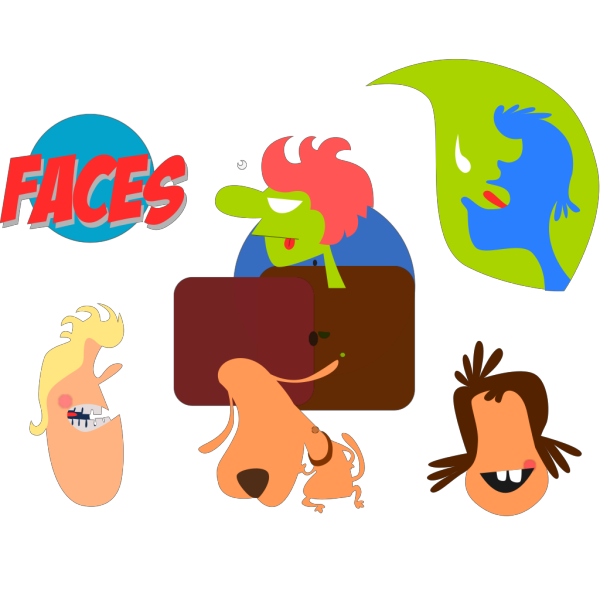This image is a collection of digital cartoon drawings set against a white background. Dominating the top left corner is a blue circle with the word "FACES" written in red ink prominently in front of it. Adjacent to this, in the top right corner, is a blue silhouette of a human figure surrounded by green, seemingly attempting to taste a raindrop. Below it, there are six distinct cartoon drawings distributed across the image. Towards the bottom left corner, there's a jagged-toothed human silhouette with blonde hair, appearing to laugh. Centrally positioned is an animated dog, peculiar for having no eyes, but depicted in a dynamic, dance-like pose with a black nose and collar. Midway up, there's a whimsical green-skinned creature with red hair, exuding a zombie-like aura. Finally, in the bottom right corner is a character with brown hair and prominent buck teeth, also without eyes. Each figure is rendered in an exaggerated, cartoony style, with large heads and unique, quirky features.